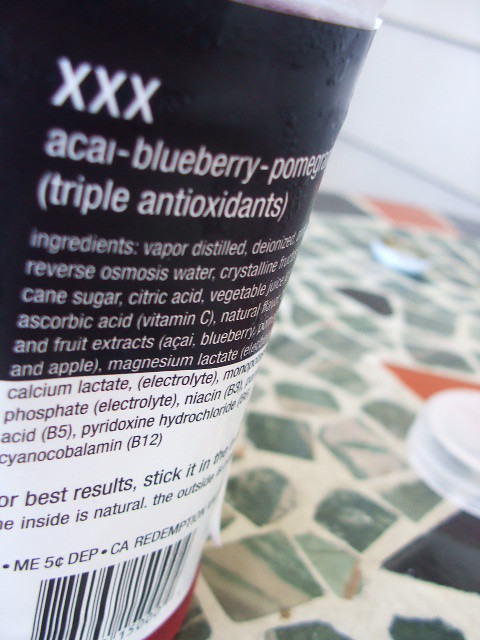The image depicts a cylindrical container of an electrolyte drink with a primarily black and white label. Prominently displayed on the label is the product name "XXX Acai Blueberry Pomegranate Triple Antioxidant," enclosed in brackets. Below this title, there is a list of ingredients, including terms such as vapor distilled water, denatured something, reverse osmosis water, crystalline cane sugar, citric acid, vegetable something, ascorbic acid (Vitamin C), natural something, and fruit extracts, including acai and blueberry, although some parts are partially obscured and unreadable. 

The label also shows a barcode at the bottom and part of the usage instructions, which suggest optimal results by sticking it into something, although the specifics are unclear. Another line mentions that the contents inside are natural, but the context remains confusing. The container rests on a multicolored surface, likely a round table adorned with an intricate pattern of colorful tiles. The overall presentation, coupled with the somewhat complex ingredient list, gives the product an uninviting allure.